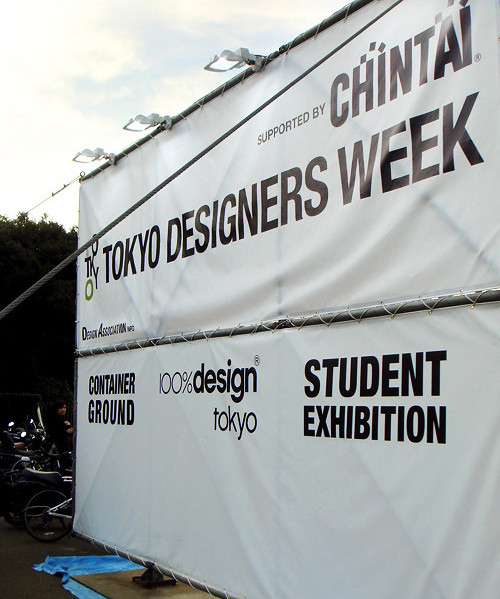The image depicts a large outdoor advertisement sign attached to a chain-link fence. The sign spans two sections of the fence and is primarily white with bold black text. At the top center, it reads "Supported by Shintai" in small black letters. Below this, across the center in large bold black letters, it states "Tokyo Designers Week". Further down, separated by a horizontal metal bar, the sign reads "Container Ground, 100% Design Tokyo, Student Exhibition". In the background, you can see a treeline and some greenery, suggesting an outdoor setting, likely taken during the daytime or around sunset given the presence of shadows and cloudy sky. There appears to be equipment, possibly motorcycles or bicycles, partially obscured by shadows. Additionally, a silhouetted figure is faintly visible, seemingly looking towards the camera. The backdrop includes patches of sky with scattered clouds, and a blue tarp is visible at the base of the sign, which stands on a concrete surface.